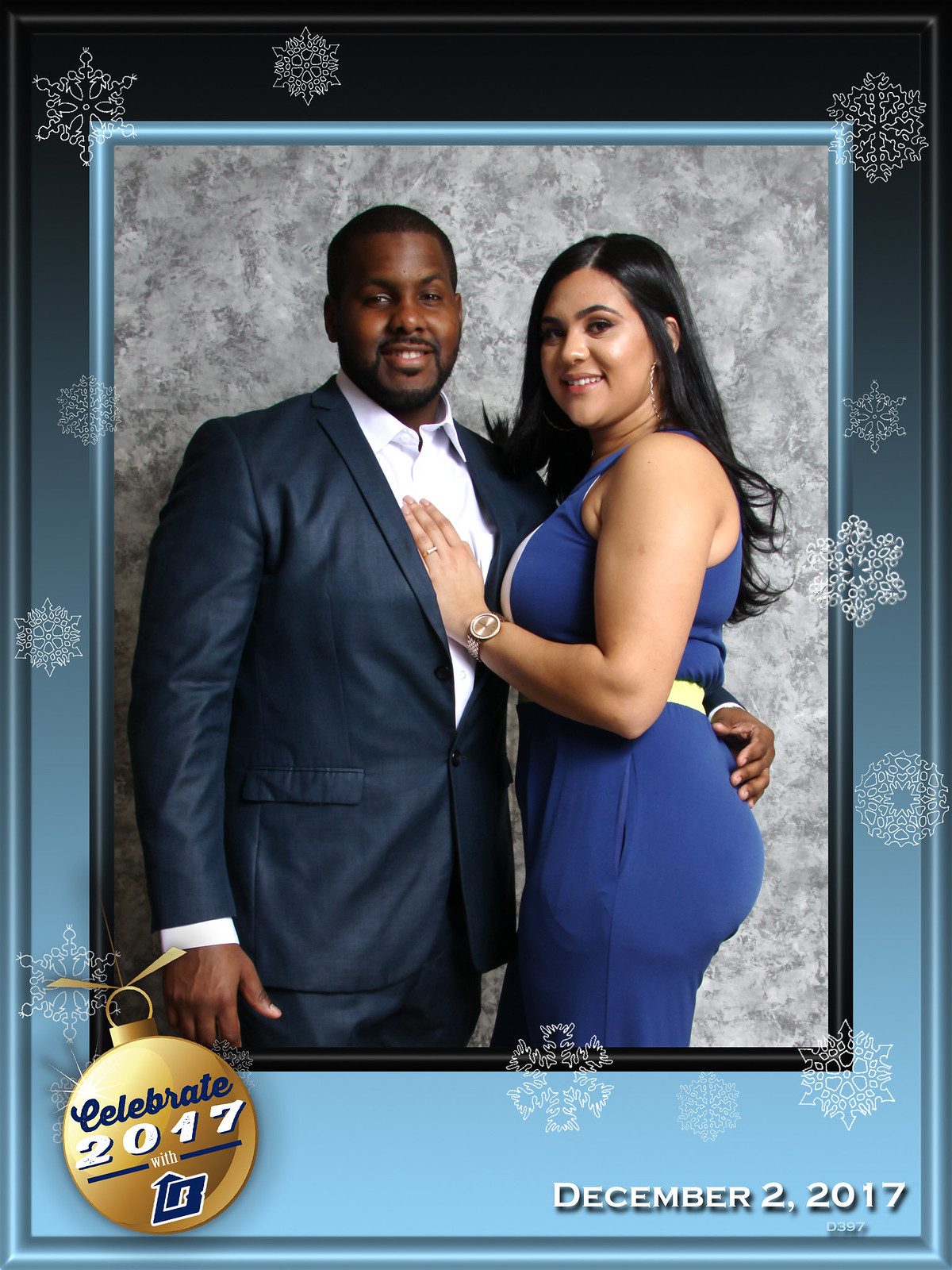The image depicts a couple posing together with a festive theme. The African American man is dressed in a navy blue suit with a white shirt, showcasing his short black hair, beard, and mustache. His arm is affectionately wrapped around a Hispanic woman with tanned skin and long black hair. She is smiling and wearing a form-fitting blue dress with a yellow belt, complemented by gold hoop earrings, a ring on her left ring finger, and a watch on her left wrist.

The photograph is bordered with a pattern of unique white snowflakes, transitioning from a black top to a light blue bottom. At the bottom left corner, there is a golden bauble ornament with the inscription "Celebrate 2017 with LB." On the right side, "December 2nd, 2017" is displayed in white text, along with the code "D397" in light blue. The overall Christmas theme is enhanced by the festive border and holiday elements.